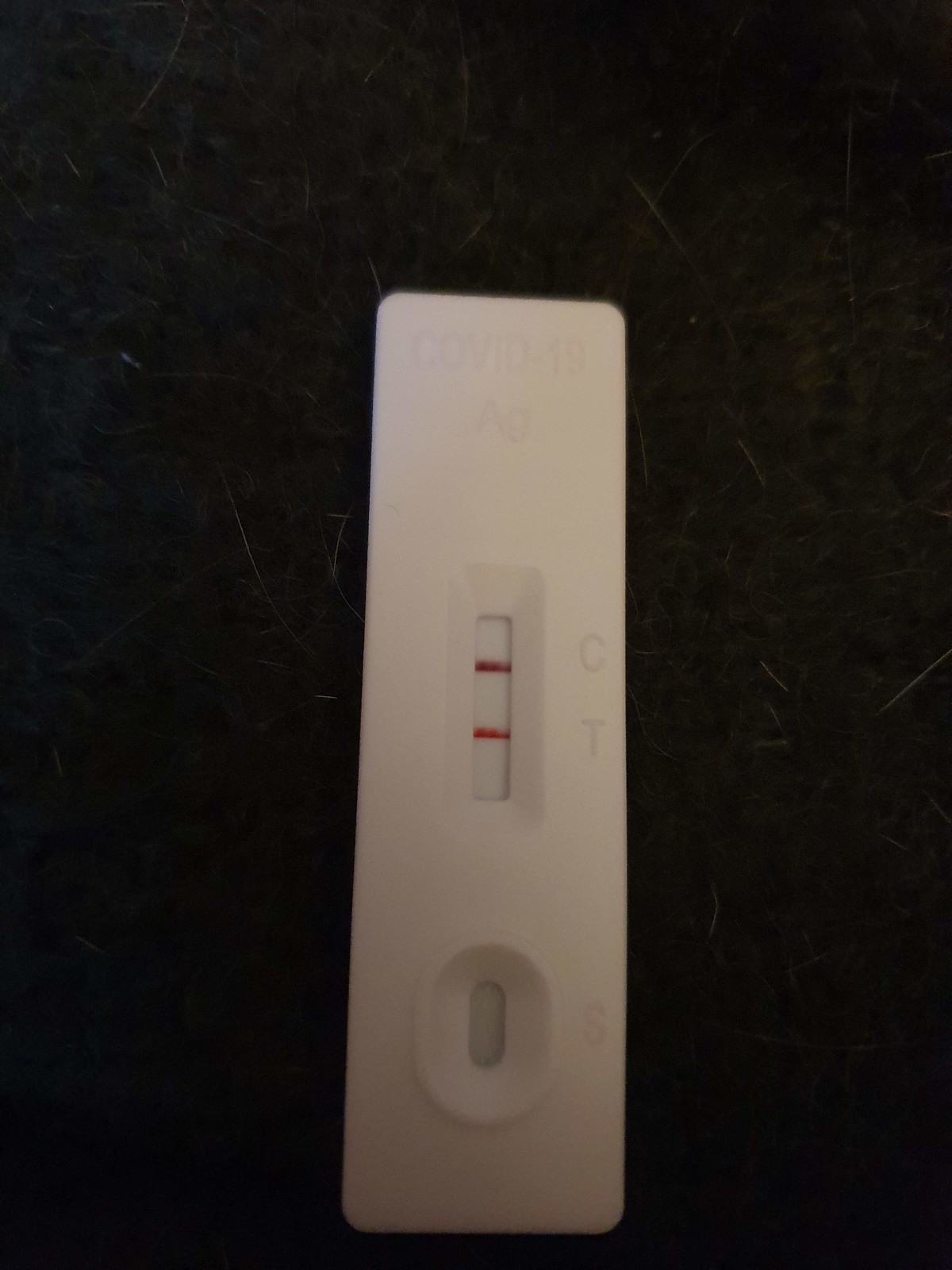A detailed close-up of a COVID-19 test kit against a solid black background. The rectangular test device, made of white plastic, prominently displays "COVID-19" etched at the top, with "Ag" (indicating antigen) written just below it. In the center of the device, there's a narrow, vertical, sunken area that houses a white view screen. On the right side of this screen are the letters "C" for control and "T" for test, each accompanied by a red line. The line next to the "C" is a darker red compared to the brighter red line next to the "T," indicating a positive result. At the bottom of the test, there is an upright, sunken oval area, which remains untouched. The image effectively showcases the design and results interpretation of a typical rapid antigen COVID-19 test.